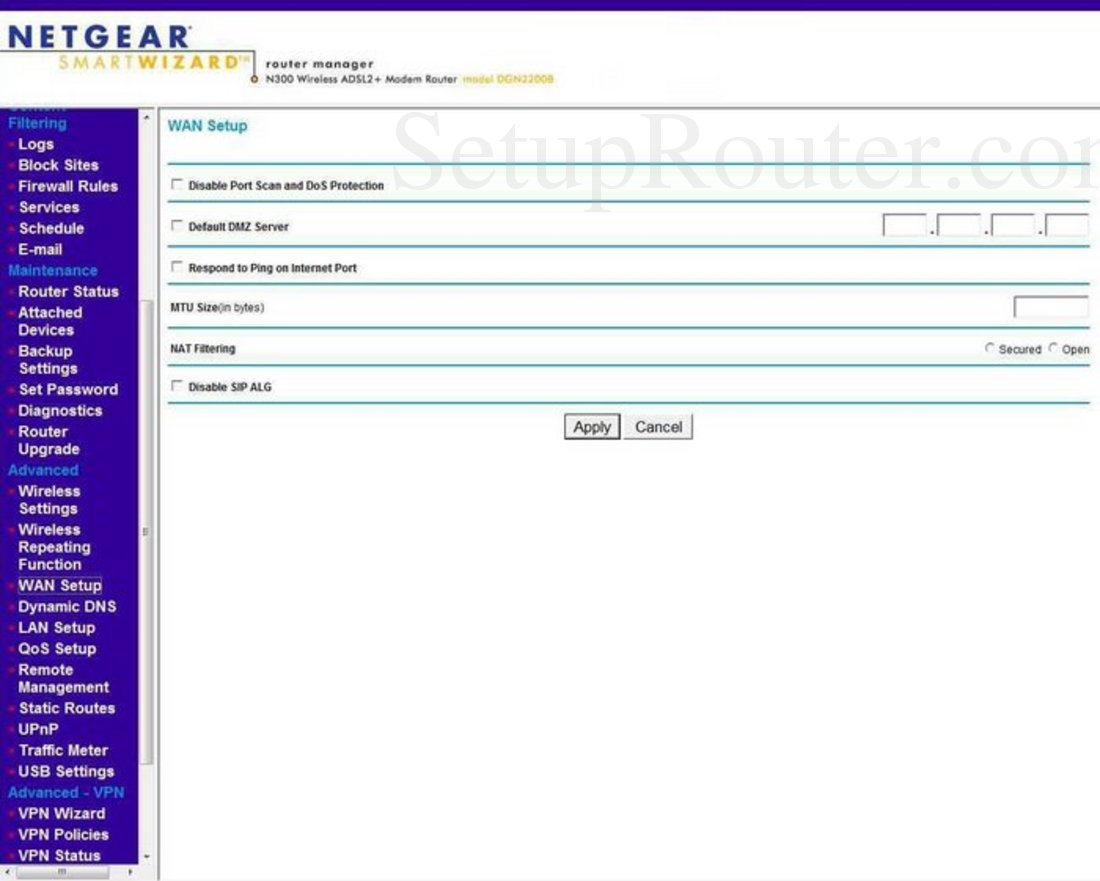This image captures a web page from Netgear's setup interface for configuring your WAN connection. The design is visually structured with a purple bar at the top, under which the Netgear logo is prominently displayed in a blue-purple hue. Below the logo, the words "Smart Wizard" appear in gold, accompanied by the phrase "Router Manager" in lowercase to the right. 

On the left-hand side, a vertical navigation column outlines various categories and subcategories against a blue and white background. The main categories include:
1. **Filtering** - with subcategories: Logs, Block Sites, Firewall Rules, Services, Schedule, Email.
2. **Maintenance** - with subcategories: Router Status, Attached Devices, Backup Settings, Set Password, Diagnostics, Router Upgrade.
3. **Advanced** - with subcategories: Wireless Settings, Wireless Repeating Function, QAN Setup (highlighted with a blue square), Dynamic DNS, LAN Setup, QoS Setup, Remote Management, Static Routers, UPnP, Traffic Meter, USB Settings.
4. **Advanced VPN** - with subcategories: VPN Wizard, VPN Policies, VPN Status.

To the right, the main content area features a grid labeled "WAN Setup" in blue, with a faint "SetupRouter.com" watermark overlay. The page presents several checkbox options and input fields for users to configure various settings. Navigation buttons located at the bottom include "Apply" (outlined in black for emphasis) and "Cancel," both in gray boxes for clear interaction points.